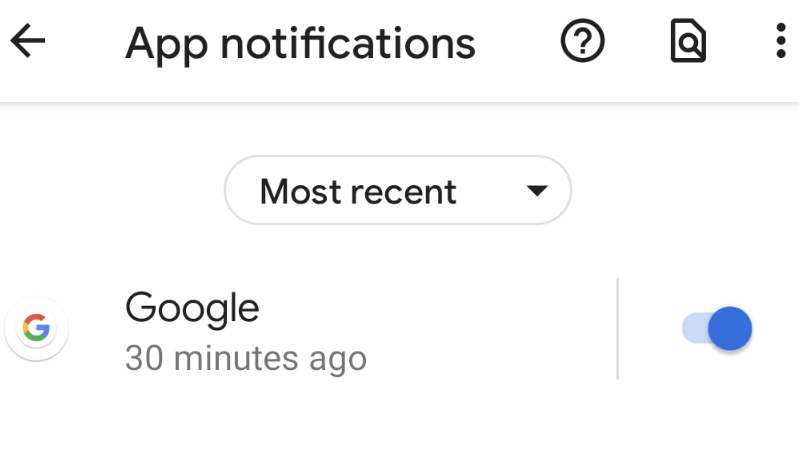This detailed cropped screenshot from a mobile phone shows a somewhat stretched and enlarged image of a section titled "App Notifications." At the top of the image, on the left, there is a left-pointing arrow. To the immediate right of the "App Notifications" title, there are three icons: a circle containing a question mark, a page icon with a magnifying glass overlay, and a menu icon. 

Below this header, in the main body of the page, there's a dropdown box set to "Most recent." Situated on the left side underneath this dropdown is the recognizable Google icon, followed by the word "Google" in large black letters. Directly below "Google," in large gray letters, it reads "30 minutes ago," indicating the last notification time. To the right, there is a blue toggle switch set to the "on" position. The screenshot has been cropped to exclude both the very top and bottom of the page, focusing specifically on the "App Notifications" title and the first notification listed under it.